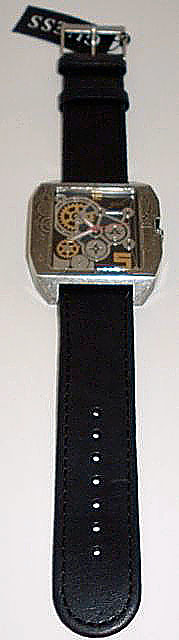In this image, a Guess brand wristwatch is displayed vertically. The black leather strap is positioned such that one end extends upwards, showcasing the metal buckle at the top, while the other end lays downward. At the center of the image, the watch face takes prominence with its intricate cog design. Despite the slight blurriness of the photo, the watch's face reveals a detailed arrangement of metallic cogs in silver and yellow tones, accentuating the sophisticated mechanical aesthetic. The label “Guess” is attached near the top, clearly indicating the brand. The image's resolution makes it challenging to discern the watch hands and finer details precisely.